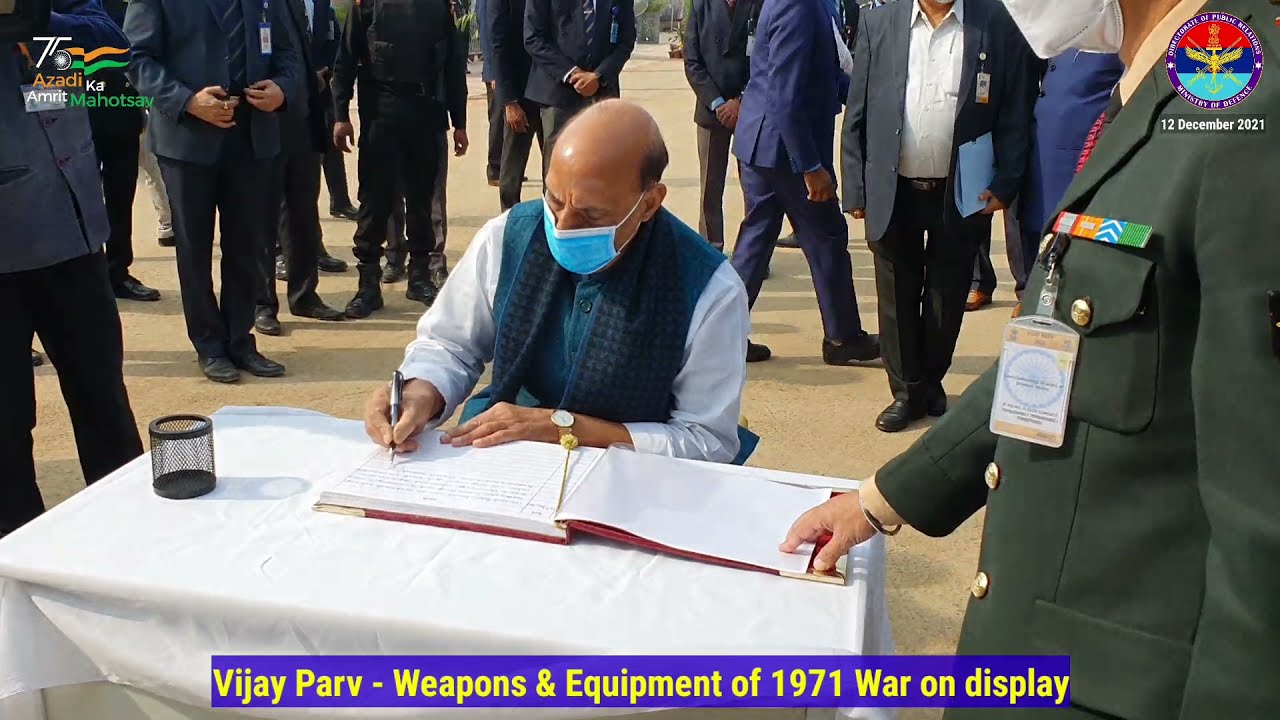In this detailed image, we observe a dark-complected man with a bald head seated at a white table outdoors, signing a red notebook with white pages using a black pen. A gold-toned watch adorns his wrist, and he's dressed in a navy blue vest, a white dress shirt, a navy blue scarf, and a face mask. The setting is bustling with activity, featuring numerous men in suits and military uniforms. Many of these servicemen, identifiable by tags and badges on their uniforms, are either holding folders or standing attentively. To the right, a man in a green military jacket holds the book open for the signer, underscoring the official nature of the event. The scene is likely from a government function or a TV broadcast, indicated by the vivid presence of various colors such as green, blue, tan, red, gold, silver, brown, peach, and white. Text at the bottom reads “V.J. Parve, Weapons and Equipment of 1971, War on Display,” overlaying a purple or bluish background. Additionally, logos with foreign letters and a date, December 2021, mark the upper corners of the image, contributing to the formality and significance of the moment.